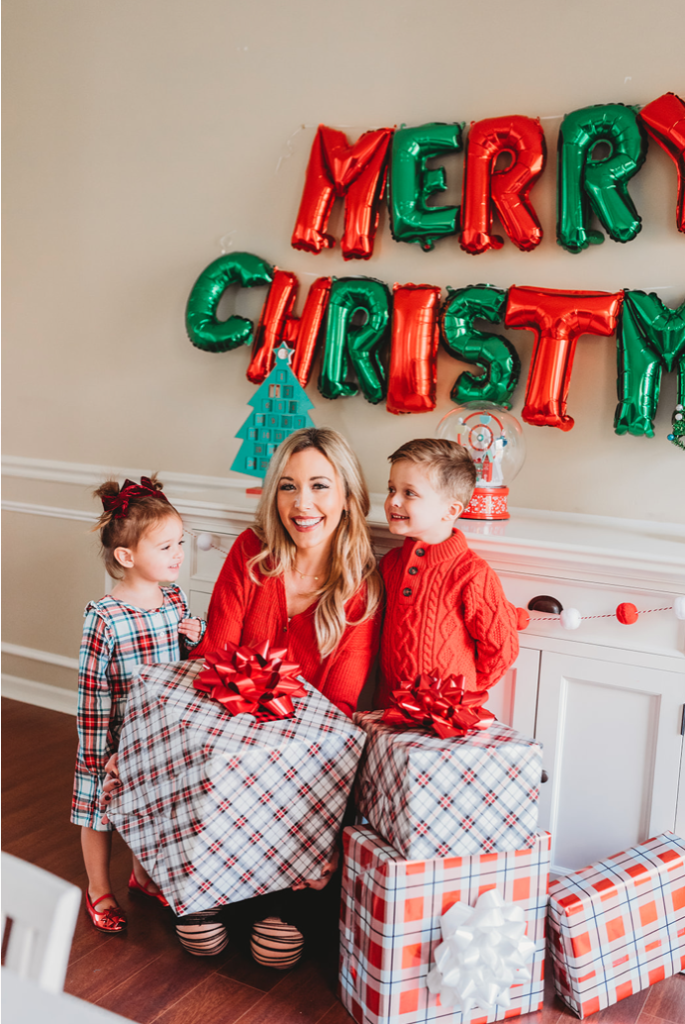In this cozy Christmas scene, a woman with long blonde hair sits on a wooden floor with her two young children, all dressed in festive pajamas and attire. The mother, in black jeans, holds a large, plaid-wrapped gift with a big red bow, while the children, radiating happiness, marvel at their own presents. The little girl wears flannel pajamas in green and red, while the boy sports a red sweater. Behind them, balloons spell out "Merry Christmas" in alternating red and green colors against an ivory-colored, cream-colored wall. Additional Christmas decorations are subtly scattered, including a tree and perhaps a globe and a banister adorned with festive accents. The overall scene captures a joyful, intimate holiday moment.